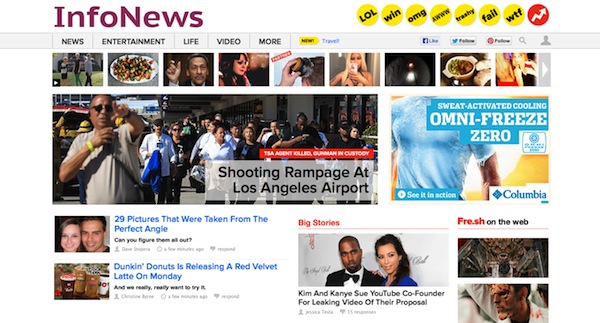This image, taken from a site called Info News, features the site's name in a reddish-burgundy print at the top. Below the title, aligned to the right, is a series of nearly all yellow circular icons with text inside them: "LOL," "OMG," "AWWW," "Trashy," "Fail," "WTF," and finally, a red circle with a zigzagging arrow.

In the center of the image is the main feature: a larger photo depicting a scene of chaos at Los Angeles Airport. In this photo, people appear to be in a hurry to exit the area. A man is pointing, and there is a figure that seems to be brandishing a gun. The text accompanying this picture reads, "Shooting rampage at Los Angeles Airport," and details the incident further with, "TSA agent killed, suspect in custody." Surrounding this central image are smaller clickable pictures presumably leading to other articles.